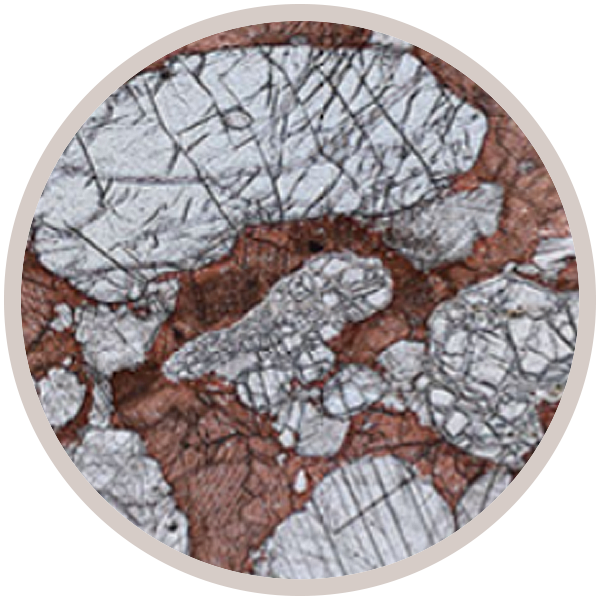This image presents a circular artwork encased in a white border, resembling a natural formation or an abstract depiction of minerals and petrified wood. The central focus features a combination of brown and gray colors, resembling fragmented shapes that could be mistaken for mineral deposits or the intricate rings of a tree embedded within the brown areas. The gray sections dominate the top portion, characterized by smoother, rounded shapes, while the brown sections at the bottom are composed of smaller, jagged fragments. Black lines run throughout the design, adding a dimensional feel and segmenting the different areas of the rocks. Despite some blurriness in the picture, the overall composition conveys an impression of a cross-section of a mineral or petrified wood, emphasizing its layered, textured appearance.